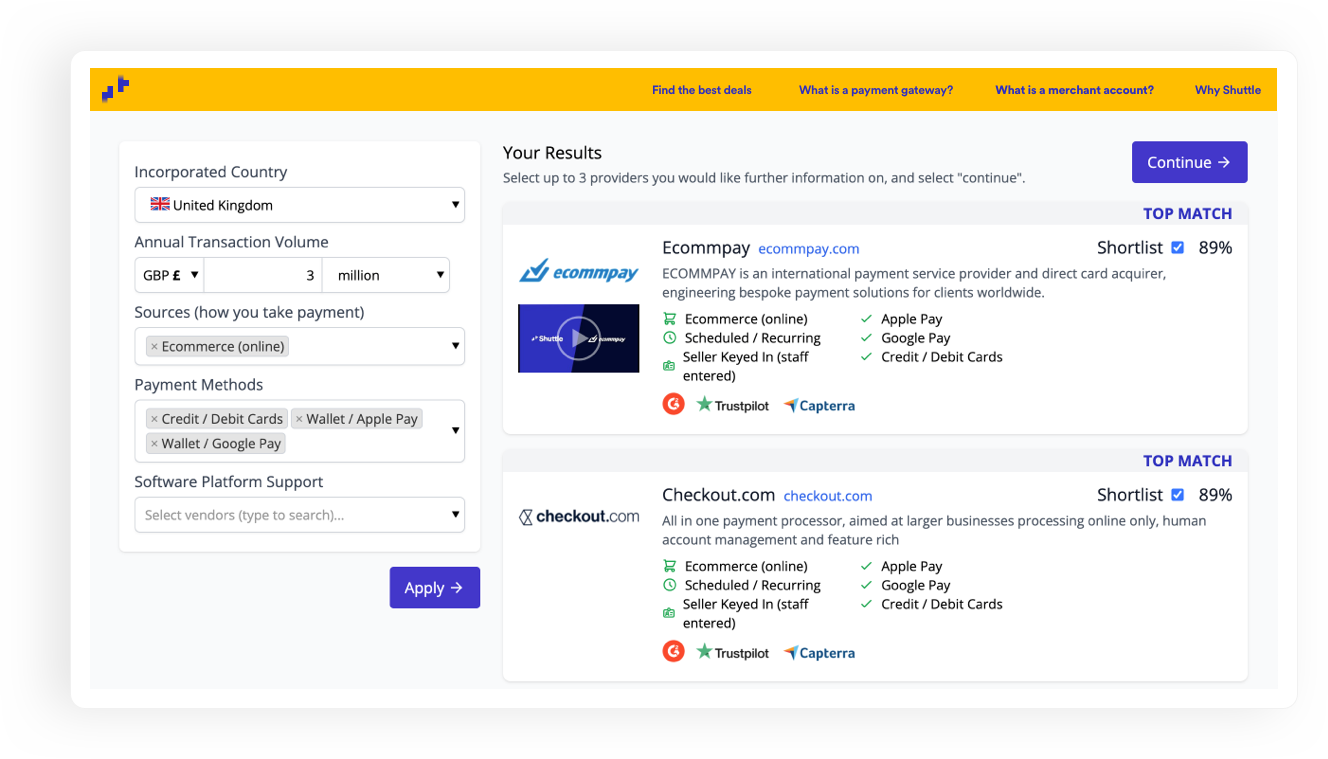The image shows a sophisticated, user-friendly section of a financial service comparison website, designed to help businesses find and select the best payment gateway and merchant account services. The webpage features a gold band across the top, with a blue text prominently displayed from the middle to the right side reading, "Find the best deals." Below that, the main section of the form is presented on a clean white background.

The left side of the form includes a series of dropdowns and input fields:
- "Incorporated Country": A dropdown menu with "United Kingdom" selected.
- "Annual Transaction Volume": A field where "GPB" and the pound sign are displayed, followed by two dropdowns showing "3" and "million," respectively.
- "Sources": A dropdown where "How do you take payment?" is specified as "E-commerce online."
- "Payment Methods": Multiple options are listed including "Credit Card," "Debit Card," "Wallet Apple Pay," and "Wallet Google Pay," with an indication there are more options available via a dropdown.
- "Software Platform": A dropdown menu to "Select Vendors," and a search bar to type and find specific platforms.
- "Apply": A button for submitting the form.

Occupying more than half of the right side of the image is the results area, which states, "Select up to three providers you would like further information on and select continue." A prominent blue button labeled "Continue" is also shown. One highlighted option in the results list is "epay.com," described as "Epay is an international payment service provider and direct card acquirer, engineering bespoke payment solutions for clients worldwide."

This detailed depiction emphasizes the webpage's comprehensive options and user-centric design intended to streamline the process of selecting financial service providers.